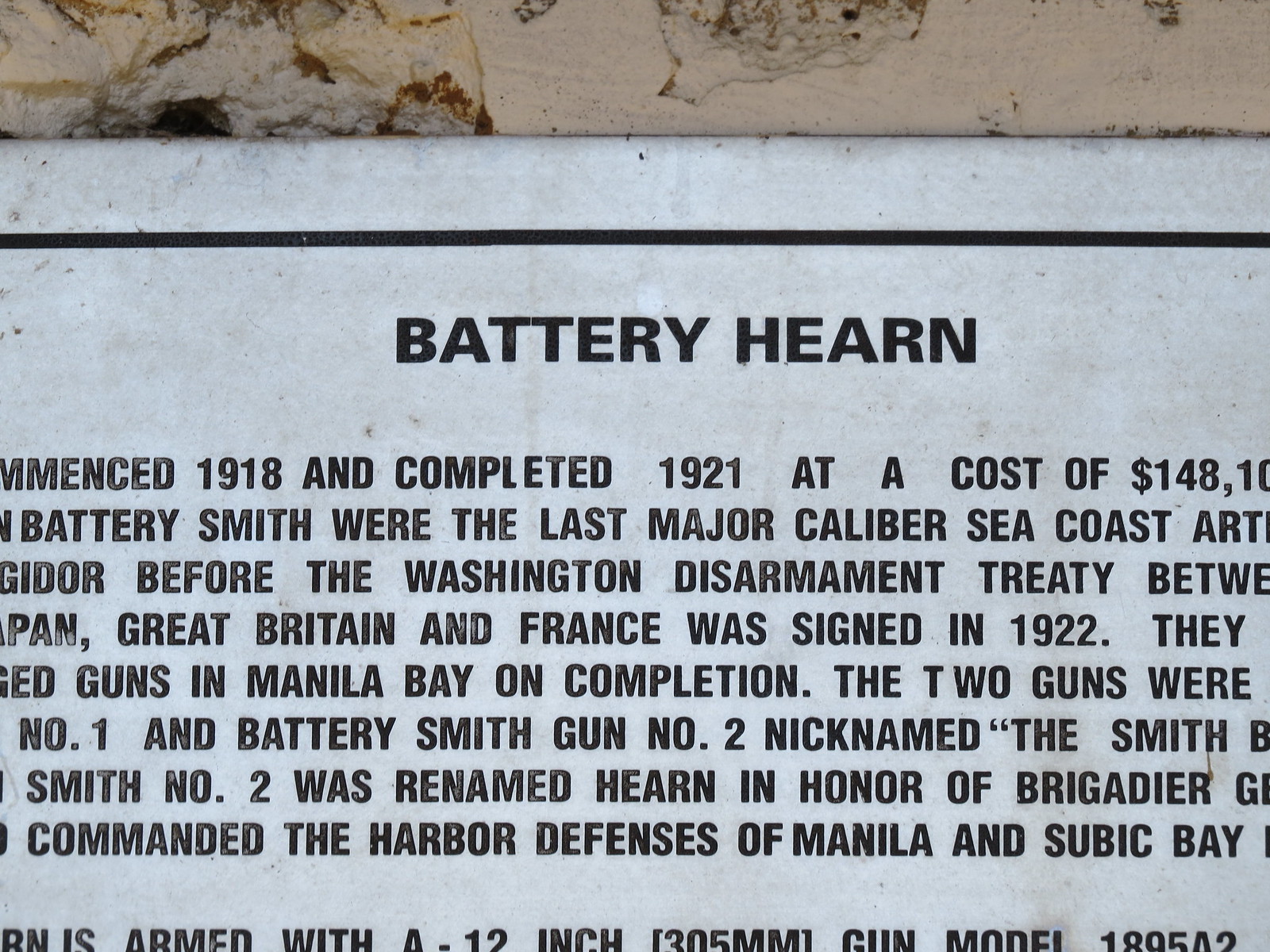The image depicts a white metal sign with a black pinstripe border across the top, set against a blue background with a concrete wall that has a worn, chipped pink surface with white and brown accents. The sign, which appears to be cut out from a newspaper, features bold black text stating "Battery Hearn." Below that, the partially visible text reads: "Commenced 1918 and Completed 1921 at a cost of $148,010." The incomplete lines go on to mention "Battery Smith were the last major Caliber Seacoast Artillery before the Washington Disarmament Treaty in 1922 between Japan, Great Britain, and France." There are references to "guns in Manila Bay" and "completion of the two guns, number one and Battery Smith gun number two, nicknamed the Smith B." Further text notes that "Smith number two was renamed Hearn in honor of Brigadier G., who commanded the Harbor Defenses of Manila and Subic Bay." The sign, framed by the rough, textured wall, holds historical significance, hinting at the military history associated with Battery Hearn.